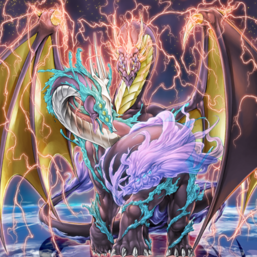This is a highly detailed digital artwork depicting a fantastical scene centered on a large, unfriendly, multicolored dragon with a mint green body and a white underbelly. The dragon's neck twists dramatically around its body, curving downward so its face is oriented towards the bottom right corner of the image. Outlining its formidable size, the dragon's extensive wings stretch from the top to the bottom of the frame, encompassing the entire composition. These wings, highlighted with bolts of lightning and electricity originating from the top, frame a vibrant backdrop of pink and yellow lightning strikes. The dragon stands on a stone pedestal, enveloped in cascading hues of purple and turquoise light that accentuate its fearsome demeanor. The ground beneath suggests a shimmering expanse of blue, gray, and white water, adding to the mystical atmosphere of this cartoony yet imposing scene.